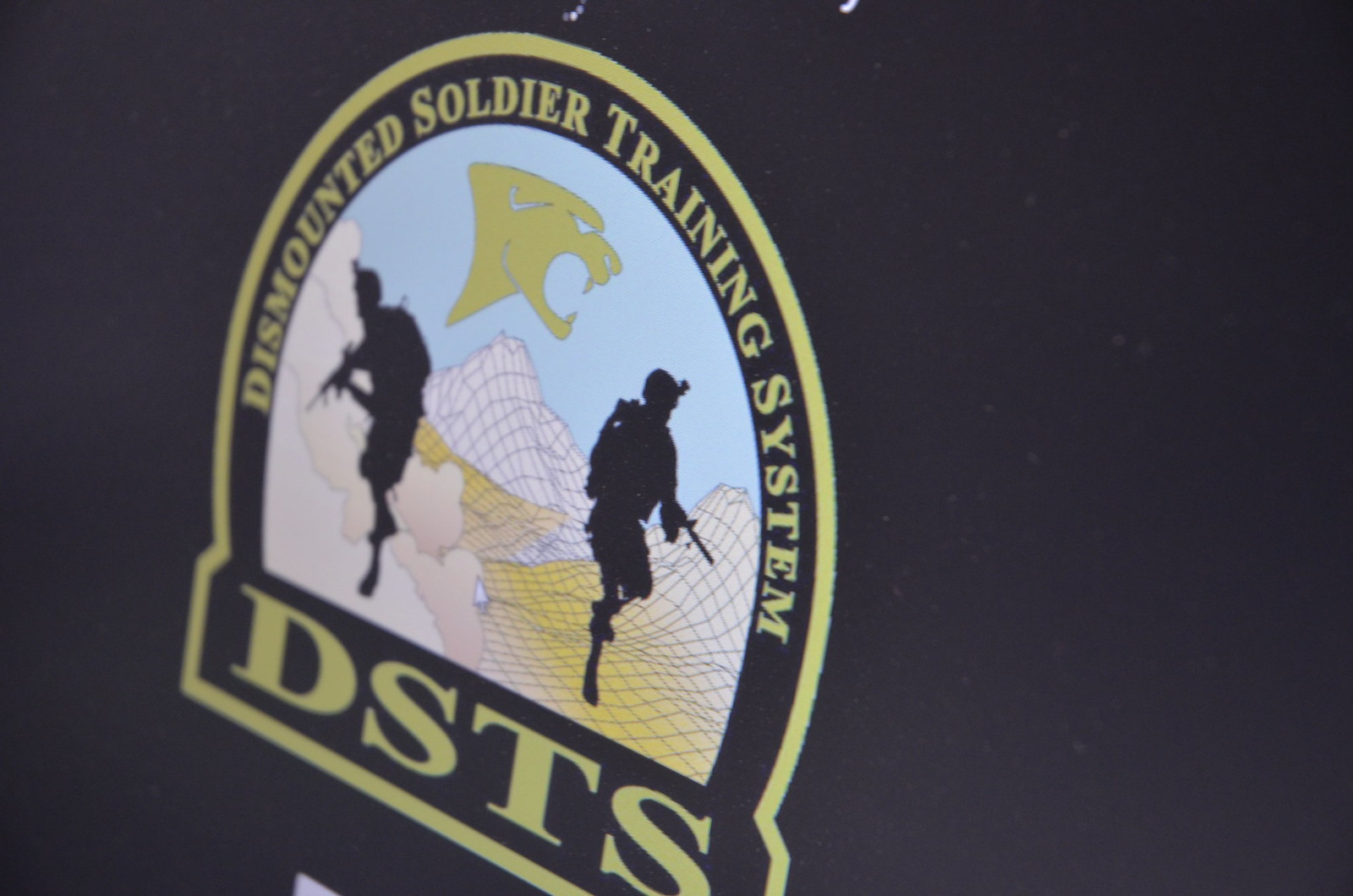This is a detailed close-up photograph of an embroidered badge, slightly angled to the bottom left. The badge is set against what appears to be a dark blue, nylon-like shirt. The badge itself is primarily circular, transitioning into a rectangular base at the bottom quarter. Encircling this badge are two gold outlines, creating both the outer and inner circular boundaries. In the inner section of the badge, the dark blue or black field hosts a graphic depiction of a tactical map, showcasing a 3D multi-line rendering of a desert-like terrain with mountains. Positioned on this map are two fully equipped soldier silhouettes, one facing left and the other right, both holding weapons. High above them, a roaring yellow jaguar or cougar with a triangular eye is prominently displayed, its mouth open to reveal both top and bottom teeth. Surrounding this central imagery, in curved gold lettering, are the words "Dismounted Soldier Training System." At the rectangular base of the badge, the bold serif gold initials "DSTS" (Dismounted Soldier Training System) are clearly visible.